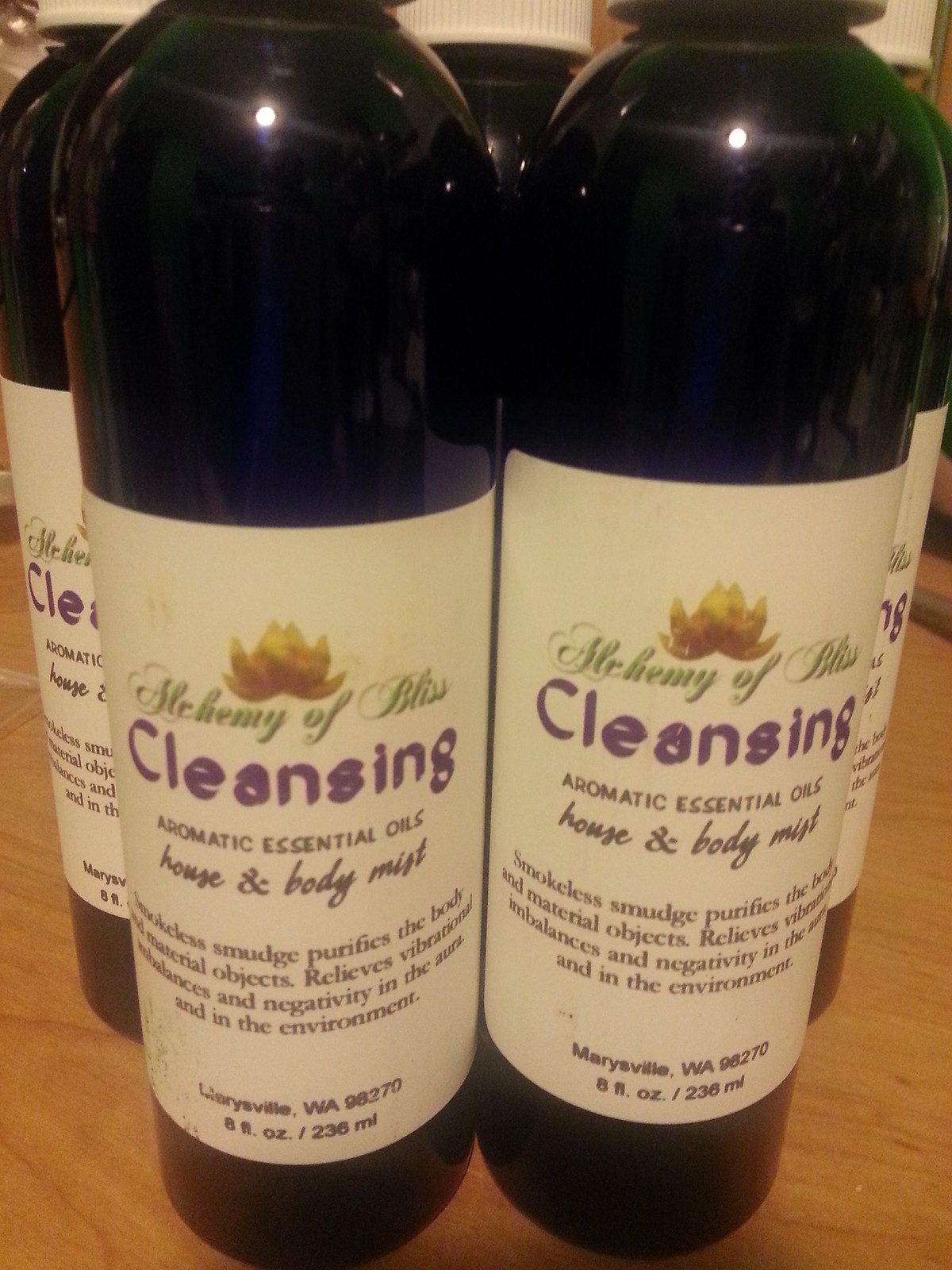This indoor, close-up color photograph captures two tall, cylinder-shaped bottles of essential oils prominently in the foreground. The bottles are dark purple and taper towards the tops, which are capped with white. The entire image is slightly grainy, emphasizing the textured wooden countertop they are seated on. The labels are beige, displaying a golden lotus flower at the top center. Wispy green cursive text reads "Alchemy of Bliss," followed by "Cleansing" in bold purple letters. Below that, in dark lettering, are the words "Aromatic Essential Oils House and Body Mist," along with a description of the mist's purpose. Other details include “Marysville, Washington 98270” and "8 fluid ounces 236 ml" at the bottom of the label. The image also reveals two more identical bottles in the background, slightly to the left and right, creating a sense of depth and continuity. Light reflections subtly highlight parts of the bottles, adding to the overall clarity and detail of the photograph.